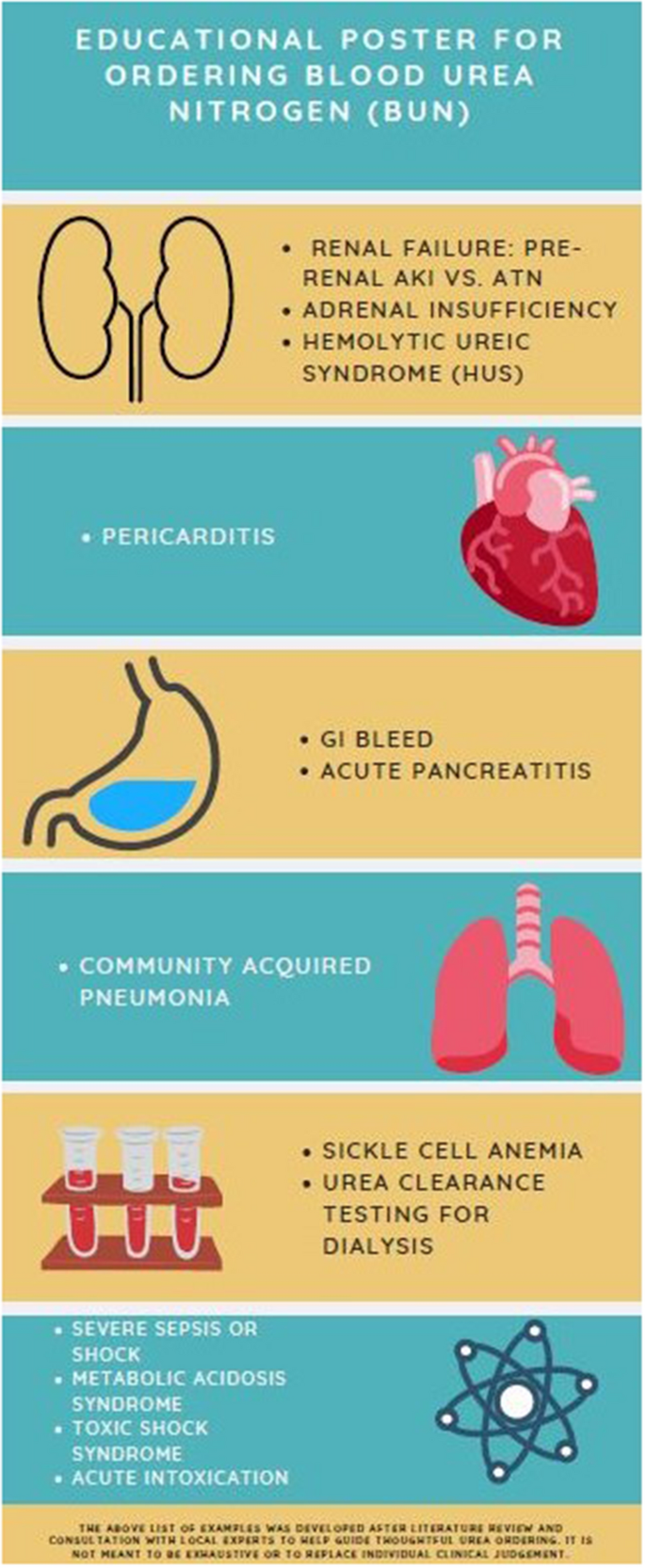The image is a vertically oriented infographic with a series of horizontal strips that alternate between blue and a yellow-orange color, separated by narrow white gaps. At the top, it’s labeled "Educational Poster for Ordering Blood Urea Nitrogen (BUN)." The poster is designed for informational purposes, likely for a hospital pamphlet or a science book, and features a mix of text and detailed illustrations.

Each strip on the poster highlights different medical conditions and symptoms associated with blood urea nitrogen levels. The top strip features a diagram of kidneys, detailing issues like renal failure and acute kidney injury (AKI). Below, a red-colored heart illustration discusses pericarditis. Further down, a stomach diagram addresses gastrointestinal (GI) bleed and acute pancreatitis. A section with lungs is labeled community-acquired pneumonia.

Next, an image of test tubes with blood talks about sickle cell anemia and urea clearance testing for dialysis. Following this, a scientific symbol represents severe sepsis or shock, metabolic acidosis syndrome, toxic shock syndrome, and acute intoxication. The overall poster uses a combination of blue and yellow-orange colors to differentiate each section, with accompanying diagrams of the heart, kidneys, stomach, and lungs, providing a comprehensive educational resource.